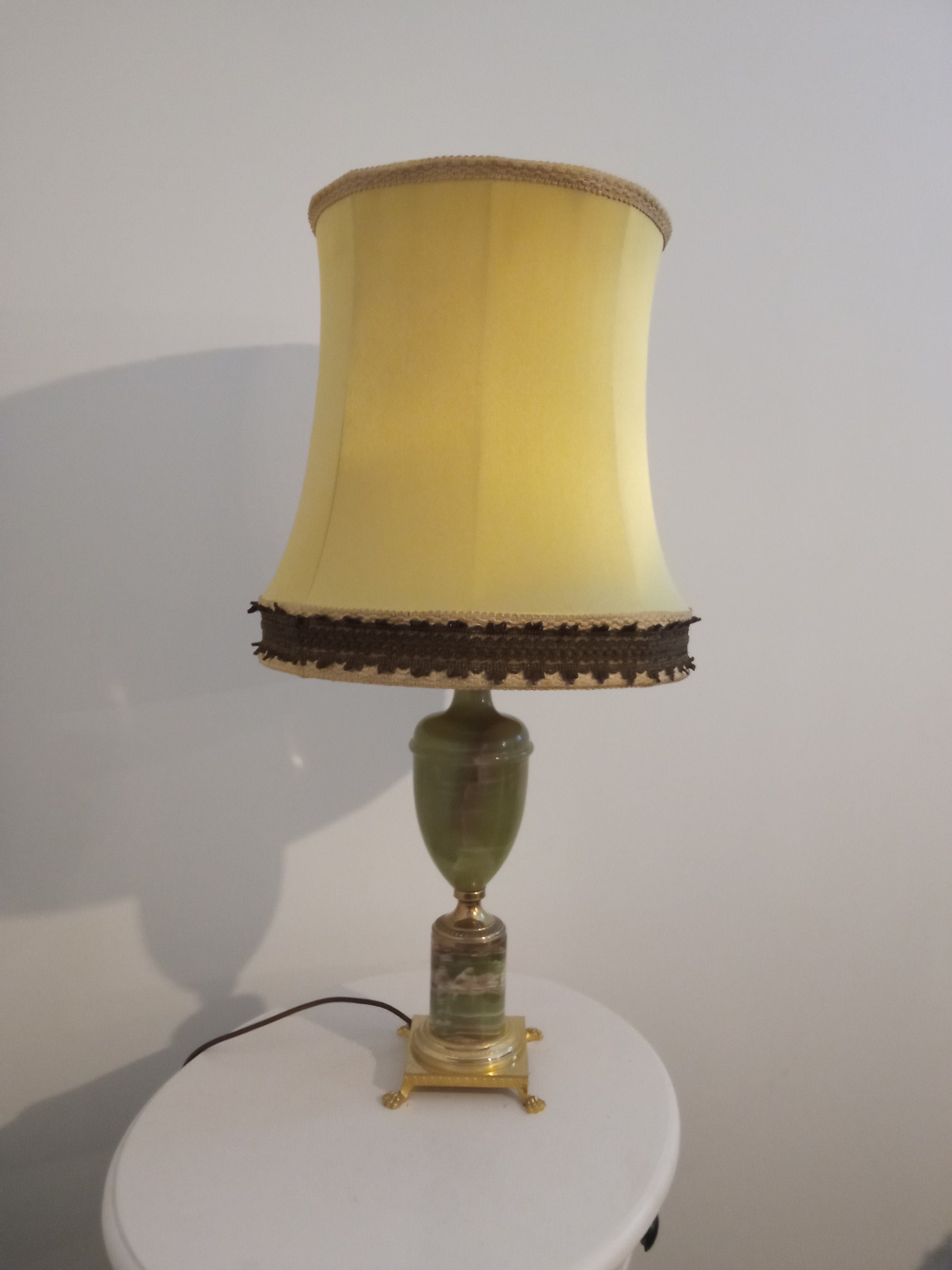The image is a detailed indoor photograph of a lamp placed on an oval white wooden table, positioned in front of an off-white or eggshell-toned wall. The camera, situated about three or four feet from the lamp, captures the lamp casting a somewhat distorted shadow to the left on the gray wall. The table surface is a small, circular-disc shape, and a brown or black electrical cord runs from the base of the lamp, trailing down past the back of the nightstand. The lamp features a square brass-colored metal base with four little feet at its corners. From there, it rises with a green cylindrical piece topped with another gold tip. The lamp's body continues with an elongated acorn-shaped structure made of green glass. The lampshade, slightly curved inward, is tan-yellowish with brown lacing running across the bottom of it.